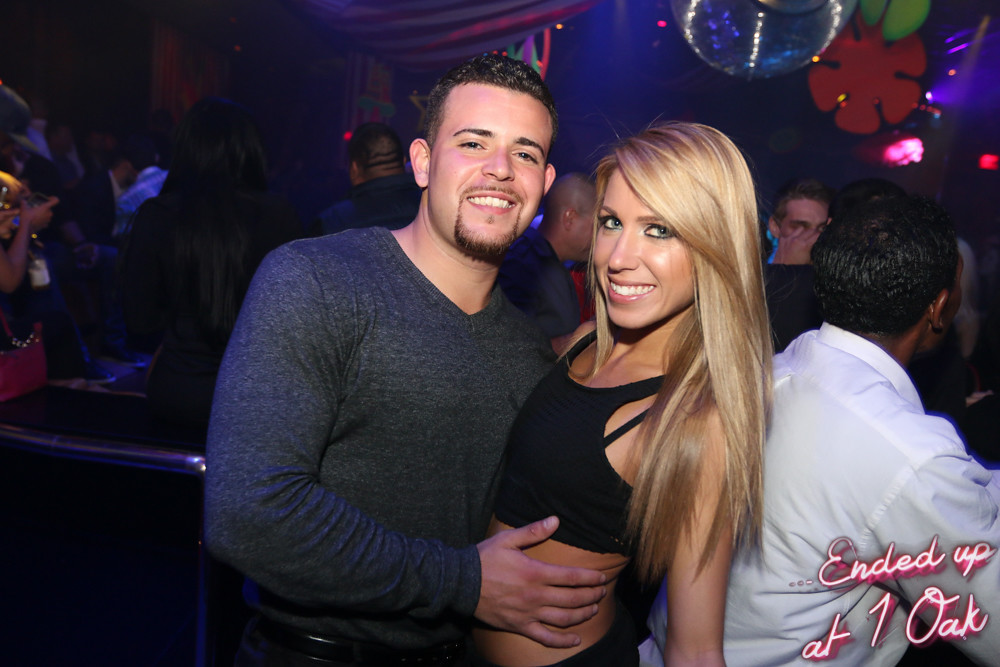In this vibrant color photograph, the focus is on a young adult man and woman at the center, illuminated by a flash or spotlight in what appears to be a darkened, bustling nightclub. The background reveals a sea of other partygoers dressed in semi-formal, stylish nightclub attire, most of whom are seen from behind, seated at tables and sipping on drinks.

The nightclub's ambiance is detailed with dark blue walls adorned with colored lights and a possible disco ball hanging from the ceiling, which adds to the festive atmosphere. In the bottom right corner, pink text reads "Ended up at One Oak," suggesting this is a promotional image for the club.

The man, with short dark hair, is dressed in a gray, long-sleeved shirt and is holding the woman affectionately close. The woman, with long dirty blonde hair, has a tan complexion and wears a short black crop top paired with black pants. Both are smiling warmly at the camera, seemingly enjoying the lively environment.

To the right of the woman, a man in a white shirt can be seen very close to her, adding to the sense of a crowded and energetic nightclub setting. The interplay of light and shadow, along with the vivid expressions and fashionable attire of the central figures, encapsulates a moment of joy and conviviality at this popular nightlife venue.